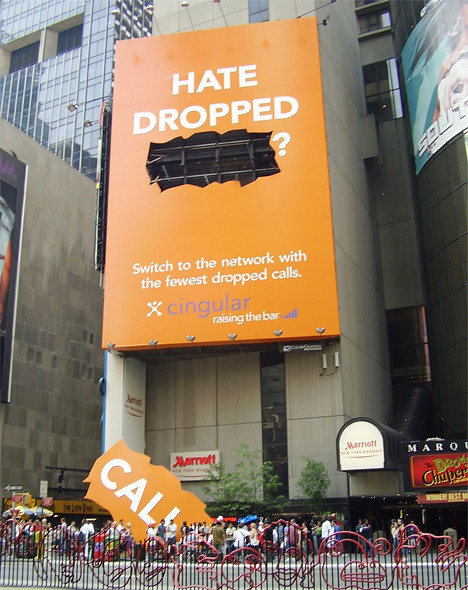In this photograph taken outside a hotel, the primary focus is a massive, vertically oriented orange billboard affixed to the side of a building. At the top of the billboard, large white letters prominently display the message, "Hate Dropped." Beneath this, a significant portion of the billboard is missing, creating a notable cutout. To the right of this cutout, there's an illustrative question mark. Directly on the ground below, the missing cutout is placed, with the word "Calls" emblazoned on it. The billboard's complete slogan reads, "Switch to the network with the fewest dropped calls. Singular. Raising the bar." Positioned beneath this towering advertisement is a sign for Marriott Hotel, indicating that the billboard is strategically located outside a hotel, likely situated in a bustling urban street.